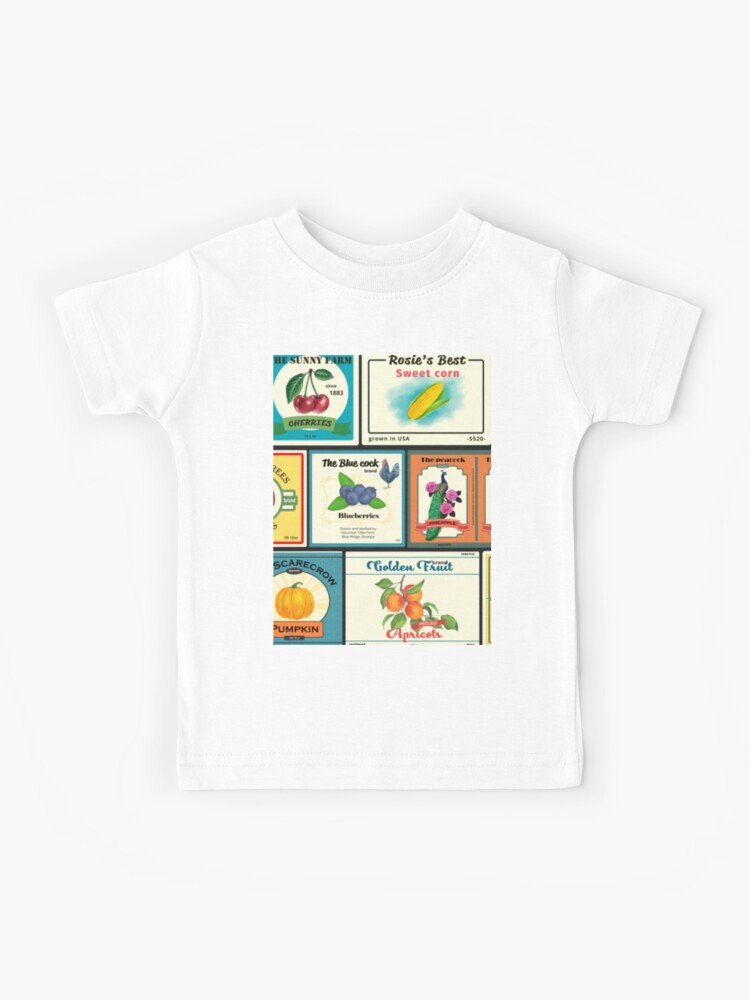The image showcases a small white child's t-shirt laying flat against a white background. This shirt features a detailed, vintage-style collage of advertisements for various farm products in the center. The design includes illustrations reminiscent of those found at farmer's markets or feed stores. At the top left, there's an ad for "Sunny Farm Cherries," depicted with vibrant cherries against a blue backdrop. Next to it, "Rosie's Best Sweet Corn" displays a bright yellow corn cob. Below, "The Blue Cock Blueberries" combines the image of a blue rooster with blueberries. Another section seems to feature cucumbers adorned with pink flowers, though it's partially obscured. On the bottom left, an ad for pumpkin reads "Scarecrow" with an orange pumpkin illustration. To the right, "Golden Fruit Apricots" shows apricots on a tree branch with green leaves. The shirt has a crew neck and short sleeves, emphasizing its simplicity and traditional form.